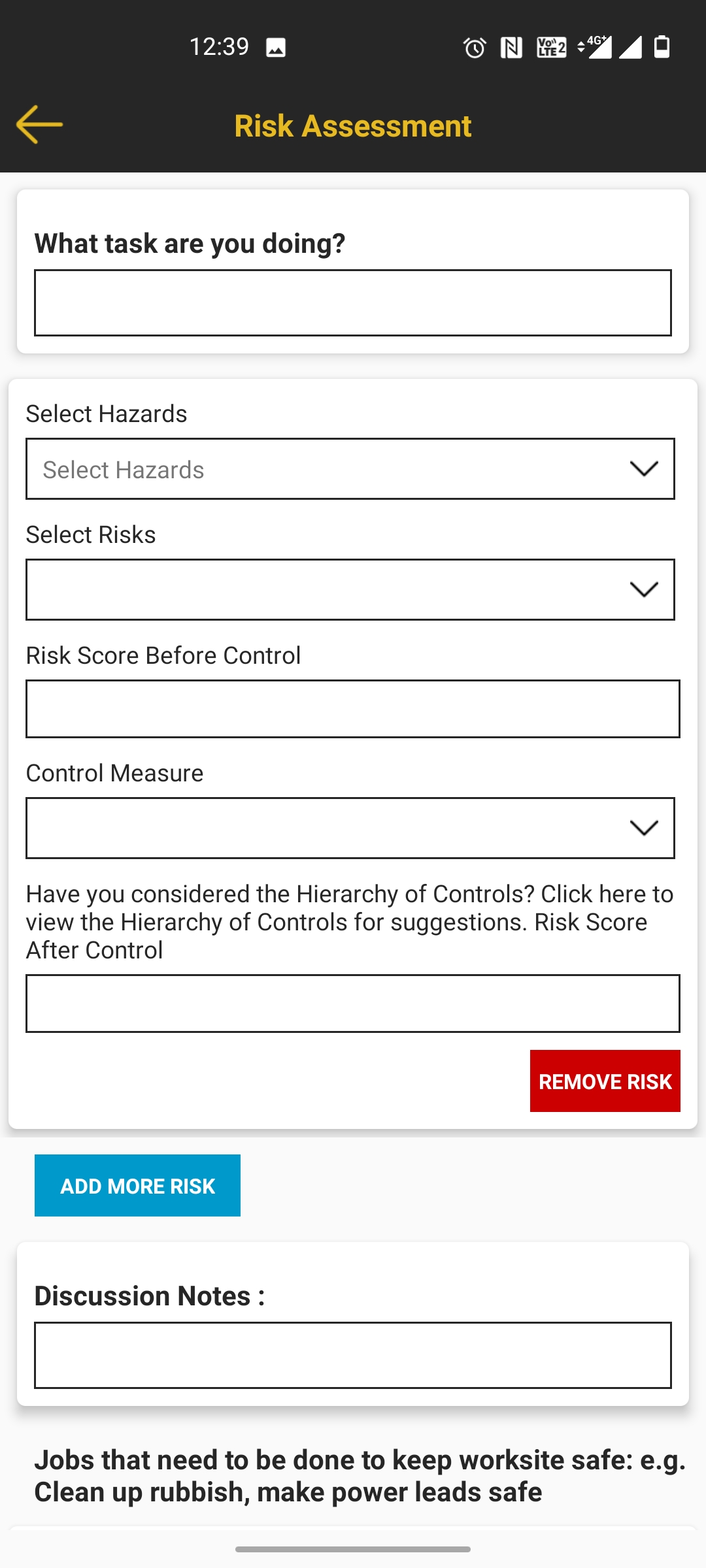Here’s a cleaned-up and detailed caption based on the provided voice description:

---

Screenshot of a mobile app interface, likely on an Android device, presented on a white background. At the top of the screen, there is a black rectangular banner stretching across the width of the device. Toward the upper right section of this banner, there are several small icons indicating the current time, battery life, signal strength, and additional notifications.

Centered at the bottom of the black banner, in yellow font, is the text "RISC Assessment." To the left of this text, there is a yellow arrow pointing backward, suggesting a back navigation option.

Below the banner, the main portion of the interface contains various input fields and options. The layout includes several white circular text boxes with instructions and fields for data entry:

1. The first section prompts the user with "What tasks are you doing?" in bold text, followed by a text box for user input.
2. Subsequently, there is a series of grouped text boxes:
    - The first box is labeled "Select tasks" and includes a dropdown menu, indicated by an arrow on the right.
    - The second box is labeled "Select RISC" which also features a dropdown menu.
    - The third box reads "RISC score before control" and includes a text box for manual entry.
    - The fourth box is labeled "Control measure" and it includes a dropdown option.
    - The final box in this group asks, "Have you considered the hierarchy of controls and other tasks?" with a text box for detailed input.

Beneath these grouped boxes, on the right side, there is a red button labeled "Remove RISC." Outside of the main white box area, at the bottom, there is a blue button labeled "Add more RISC."

Further down, a white box labeled "Discussion notes" includes a text box for additional typing. The final line on the interface, in bold, reads, "Jobs that need to be done to keep workforce safe: e.g., clean up rubbish, make power leads safe." Below this text, a thin gray line extends across the screen, not reaching the edges.

---

This detailed description provides a structured and comprehensive overview of the screenshot, encapsulating all the elements and their arrangement within the interface.